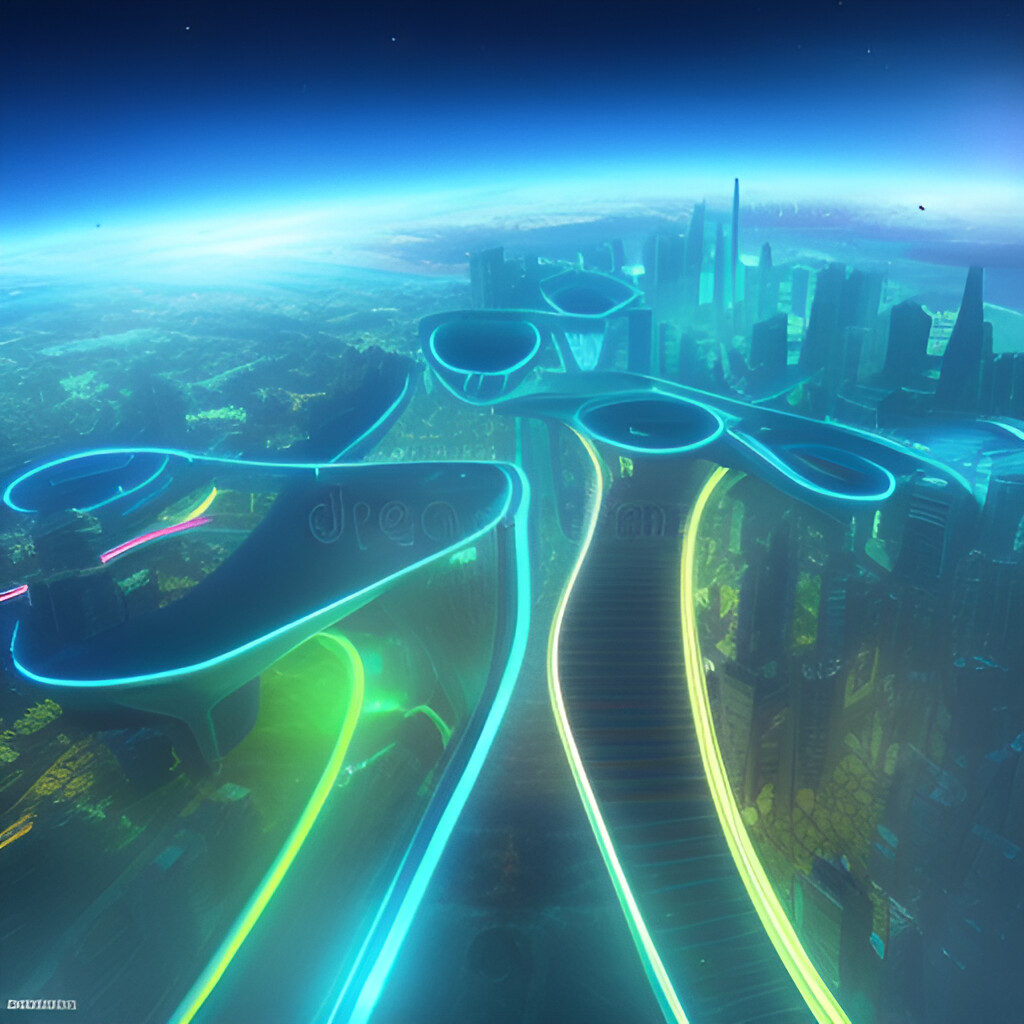The image portrays a highly detailed, computer-animated vision of a futuristic city, potentially set around the year 3000. The overall color scheme is dominated by shades of blue, giving a glowing aura to the entire cityscape, which is further illuminated with vibrant neon lights in yellow, green, and blue. 

Tall, modern skyscrapers with intricate architecture are prominently positioned to the right, while additional buildings span across the image. On the left, smaller structures are visible, accentuating the city’s layered complexity. The scene includes winding paths and streets adorned with curving, neon-lit highways, and staircases that ascend to multiple high platforms, some of which are small and circular. 

The dark blue sky contrasts against the illuminated city, enhancing the impression of a fantasy futuristic setting. There is also text in the bottom left corner of the image, written in white, though it is difficult to read. The presence of trees interspersed among the buildings adds a touch of greenery to this vivid, imaginative metropolis.